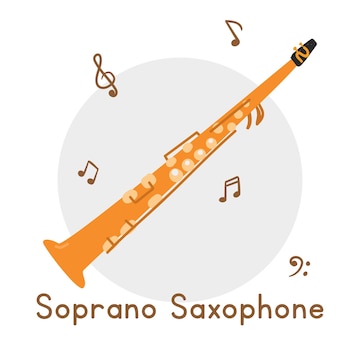This detailed illustration features a vector graphic of a golden soprano saxophone with a black mouthpiece. The saxophone starts off slender at the mouthpiece and gradually widens towards a flared bell at the end. It showcases numerous intricate details such as varied buttons for finger placement, a long skinny bar attached in two places on one side, and a smaller bar similarly attached on the other side, with two tabs near the base. A skinny bar can also be seen in the middle. Surrounding the saxophone are five brown musical notes, floating as if emanating from it, creating a dynamic visual effect. The backdrop includes a light gray circle that provides contrast to the saxophone and notes. At the bottom of the graphic, the text "soprano saxophone" is displayed in a branded brown font.